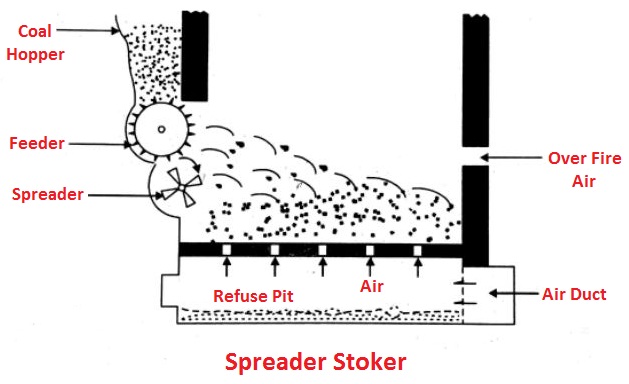The image is a detailed black-and-white diagram of a coal burning machine, labeled with text in red. At the bottom of the diagram, "Spreader Stoker" is prominently displayed in red. The labeled components include a coal hopper at the upper left, feeding coal into the feeder. The feeder directs the coal to the spreader, identified by an arrow pointing to it. Below these components is the refuse pit, again labeled with an arrow. Air flow is an essential part of the process, with arrows pointing to air, an air duct, and overfire air. Central to the diagram is a wheel, with black dots—representing coal or particles—situated on top of it. As the wheel spins, these dots are spread into the main section, where they become more numerous. The diagram focuses on outlining the flow and various components of the machine, featuring a mix of rectangles and symbols to depict the different parts and their interactions. The overall style and layout suggest it's designed for educational or instructional purposes.